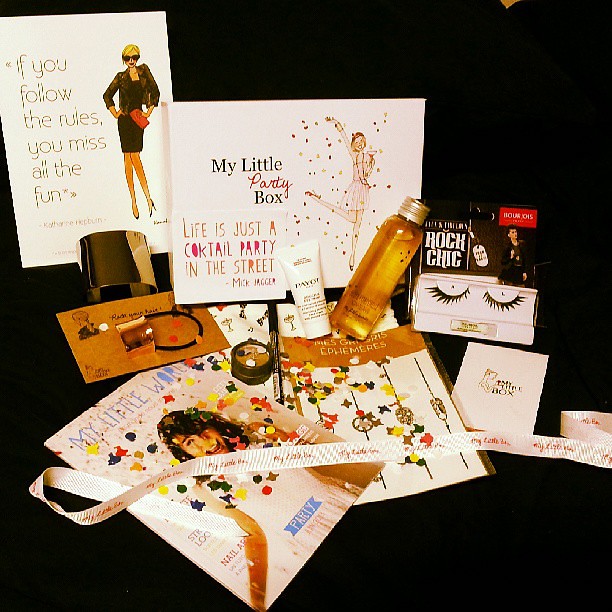The image showcases a black surface, possibly a table with a black tablecloth, spread out with various printed materials and objects, creating a vibrant and festive scene. Starting from the top left corner, there's a poster featuring a woman in a black dress with a jacket and red purse, striking a confident pose and accompanied by the caption, "If you follow the rules, you miss all the fun." To the right of this, another prominent card displays the phrase, "My Little Party Box," with the quote, "Life is just a cocktail party in the street," highlighted in red and orange, attributed to Mick Jagger. This card depicts a jubilant woman in a pink dress, with one leg bent backward and confetti swirling around her.

The central area is filled with a variety of beauty products, including a white bottle labeled "Payot" and a light tan-capped brownish bottle. Among these items, there are also a bubble bath and what appears to be body lotion or face cream. Additional beauty items include an eyeshadow, eyeliner or mascara, and a Rock Chick false eyelashes set. A potential bracelet and a couple of magazines or subscription cards, one of which might bear the recurring "My Little Party Box" branding, are also visible. A decorative ribbon ties together the ensemble, suggesting the layout might be part of a celebratory gift box geared towards a female audience. The overall scene exudes a lively and joyful atmosphere, emphasizing the theme of carefree celebration.